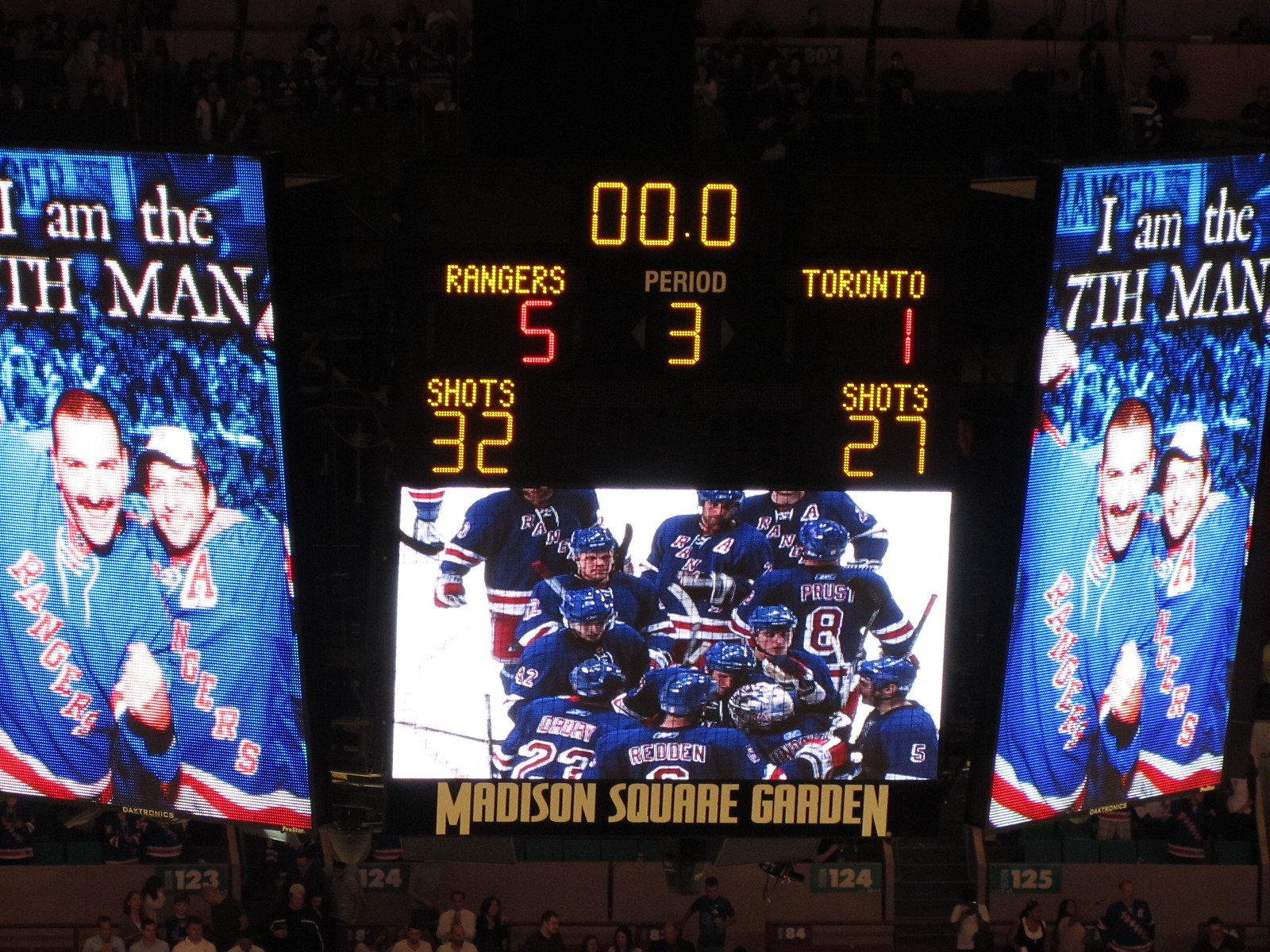This detailed photograph captures the scoreboard at a hockey game held in Madison Square Garden. The black scoreboard, viewable from multiple sides within the arena, announces the end of the third period with a final score of New York Rangers 5, Toronto 1. It also displays the number of shots on goal for each team, 32 for the Rangers and 27 for Toronto. Prominently featured on the video screens on either side of the scoreboard are the words "I am the seventh man." Below these words, images of two enthusiastic Rangers fans, both dressed in blue and red Rangers jerseys, are shown. One of the fans is wearing a baseball cap. Central on the scoreboard, a visual shows multiple Rangers players on the ice, reflecting the victorious atmosphere. The arena's signature sign, "Madison Square Garden," is visible in yellow below the scoreboard, reinforcing the iconic location of the event.